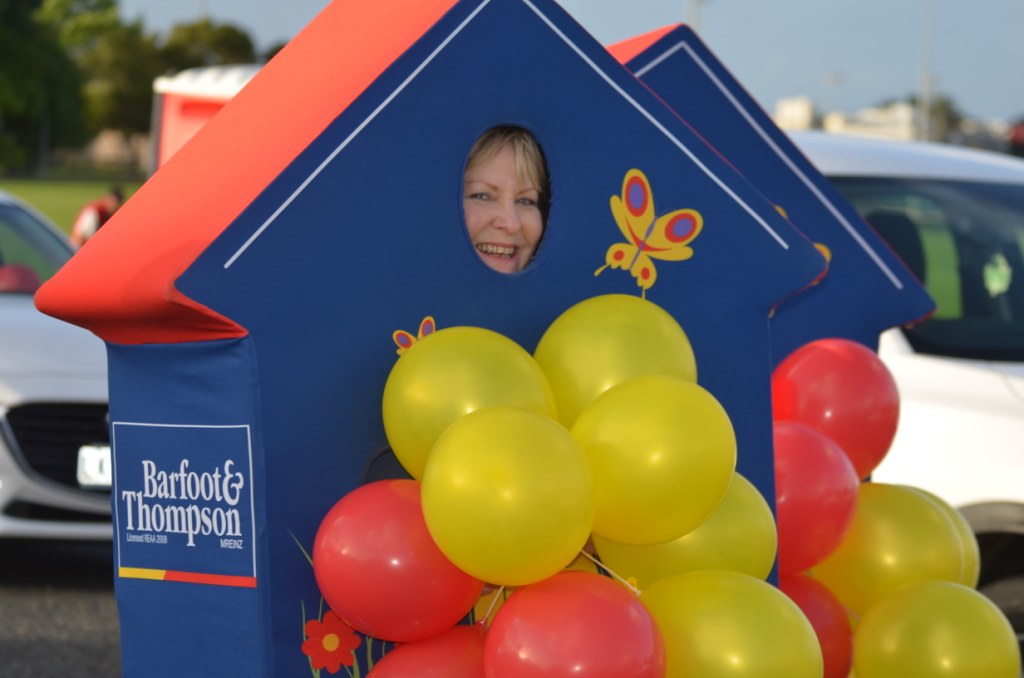In this outdoor image captured during the day, a smiling woman is at the center, dressed in a unique costume designed to look like a house. The house costume features a blue body with an orange roof and a notable hole in the upper section through which the woman's face, framed by her blonde hair, peers out. The house costume is adorned with a painted yellow and blue butterfly to the right of the woman's face, and it bears the white text "Barfoot and Thompson" on its left side. 

In front of the house costume, several colorful balloons, in shades of yellow and pink, add a festive touch. Additional yellow and pink balloons are visible to the right, further complementing the scene. The background showcases a large, grassy field bordered by trees in the upper left corner and buildings in the upper right. The setting also includes a stretch of asphalt road with blurred cars situated on either side of the image, adding to the busy yet vibrant atmosphere. The sky above completes the daytime outdoor setting, providing a clear and expansive backdrop to this cheerful and whimsical scene.